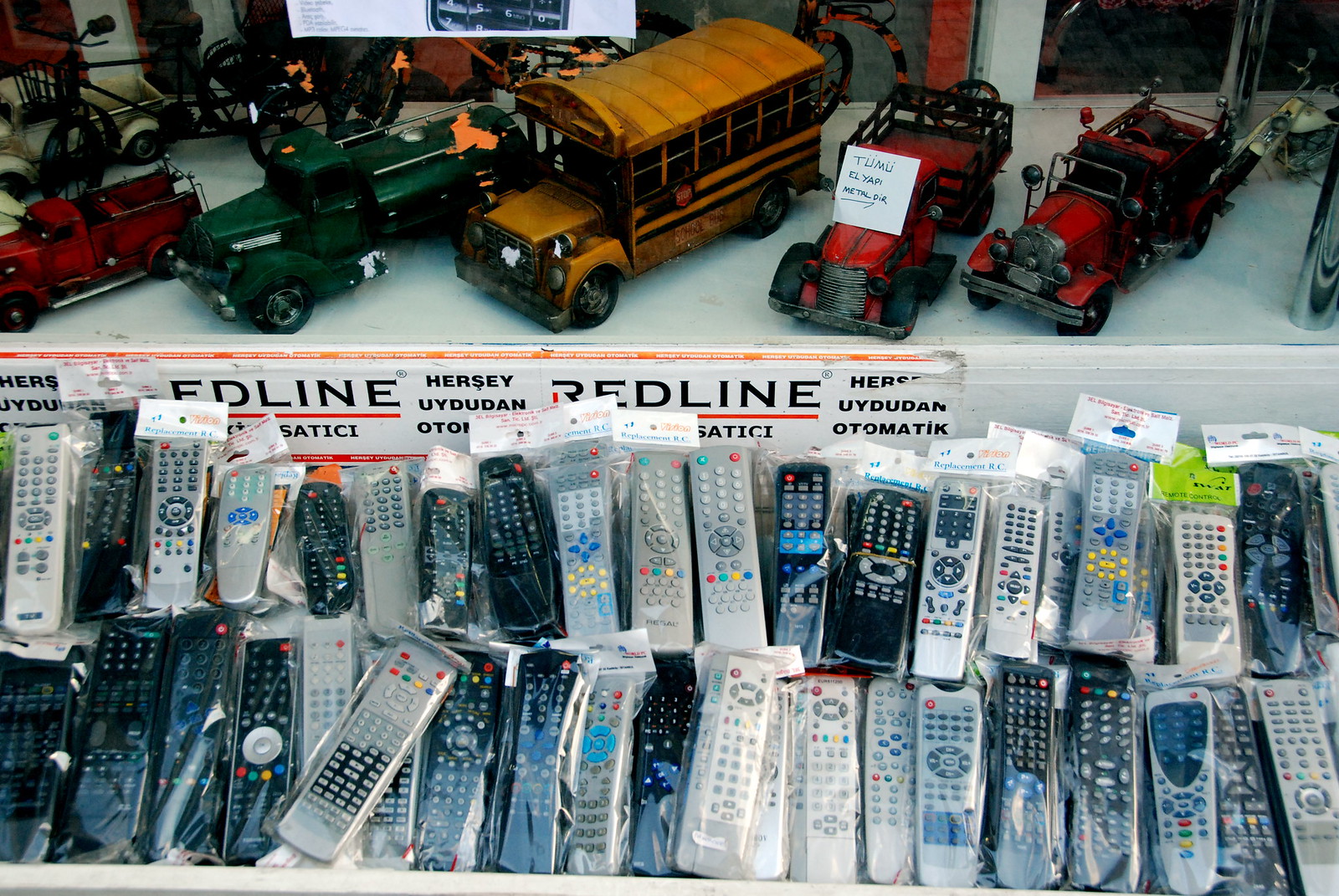The image depicts a flea market or resale shop with two shelves. The top shelf is flat and showcases a collection of older model toy vehicles, including a dirty yellow school bus, a green army truck, a red fire engine, and various other vintage trucks. The vehicles feature orange price stickers, and a white card with writing and numbers is placed on the hood of the green tractor. The second, angled shelf is densely packed with an array of remote controls, stacked from left to right. These remote controls, in predominantly grey with a few black ones, are neatly organized in plastic bags with white tags at the top. Additionally, there is a sign taped above the remotes that reads "Red Line," though the language on the sign includes words like "Jose Olladudan" that are not in English.